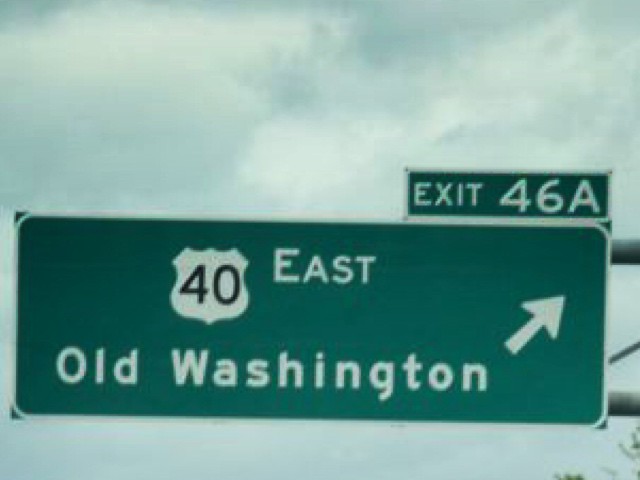A daytime photograph captures a green highway sign viewed from below, against an overcast sky filled with clouds. The sign prominently displays "Exit 46A" at the top. Below that, in large capital letters, "40 EAST" is clearly visible, with an icon encircling the number 40. Further down, the sign indicates directions to "Old Washington," accompanied by an arrow pointing to the right. The sign is the kind typically suspended over a highway, and the image is tightly cropped, focusing primarily on the sign along with a small portion of a tree's branches appearing at the bottom right.